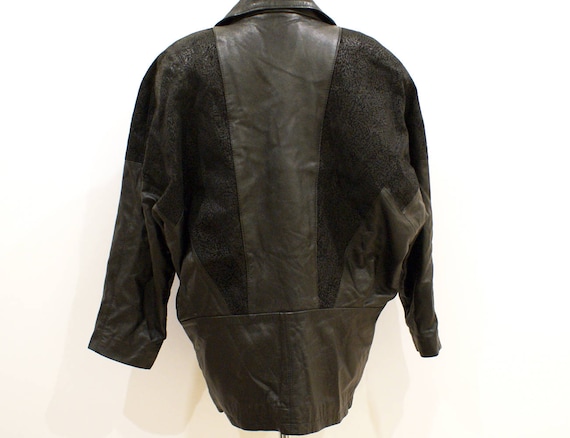The image depicts the back view of a black leather jacket, suspended against a light, creamy white background. The jacket features a distinct design with a central vertical panel made of a different material, likely a combination of smooth, shinier leather and softer, suede-like leather. The middle strip, which runs from the neckline down to the bottom, and the lower part of the jacket have a darker, almost black appearance. The rest of the jacket maintains a rich, deep black hue, contributing to a masculine aesthetic. The full-length sleeves, the absence of visible fasteners, and the back-only angle make it challenging to determine whether the jacket has a zipper or buttons. The jacket is not being worn or hung up, and no brand or style information is available, emphasizing its simple yet unique design. In the backdrop, there is a faint, barely noticeable outline of what might be another white jacket or an element of the background design, adding to the image's intrigue.